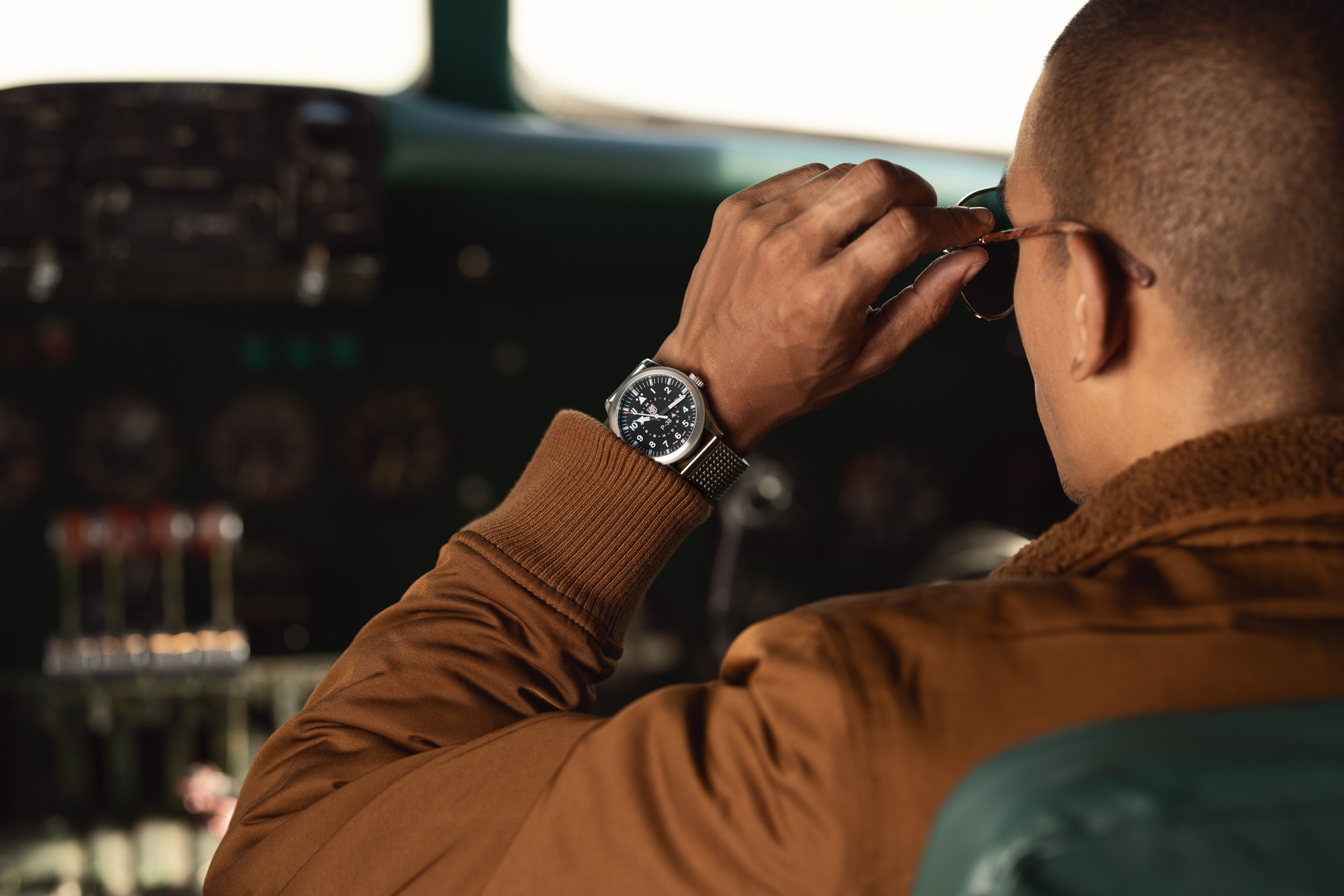This photograph captures the back left profile of a man sitting in the cockpit of an airplane. He has light brown skin and his hair is shaved very short, almost to the scalp. He wears black tortoiseshell-frame sunglasses and a silver watch on his left wrist, which is raised as if he might be adjusting or removing his sunglasses. The man is dressed in a brown jacket with a fleece collar and is seated in a grayish-green leather chair. In the background, the airplane's dashboard is visible with various dials, knobs, and a throttle on the lower left side. A split-screen windscreen is situated above the control panel, giving a hint of the sky beyond.